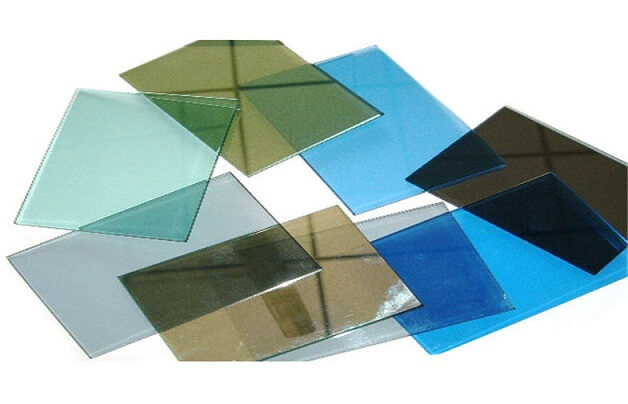This meticulously arranged image on a white or translucent background features an assortment of eight pieces of glass material, each seemingly meticulously photoshopped for clarity. The assembly includes a combination of small mirrors and tinted glass or plastic squares, which seamlessly overlap one another creating a layered composition. Among them are two clear glass sheets, a light blue piece, a medium blue piece, and a lighter blue piece with a slight tint. The image also showcases at least two conventional mirrors and a darker, almost gray mirrored piece with a subdued reflection, distinctly less polished than the others. The elements are strategically placed with some turned at different angles, enhancing their reflective and transparent properties. Notable is the lack of any dark borders or additional objects or text in the image, allowing the viewer to focus solely on the intricate interplay of colors and materials. This captivating arrangement evokes a sense of abstract artistry through its careful layering and subtle chromatic variations.